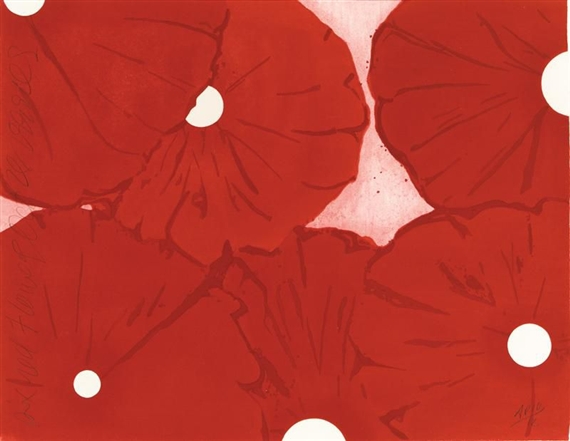This artistic painting illustrates an abstract representation of six red flowers, reminiscent of poppies, with overlapping, circular petals. Each flower features a perfect white circle at its center, from which dark red and lighter red streaks radiate outward, creating a vivid depiction of petals. The flowers, predominantly red with intricate red outlines emphasizing the petal structures, appear to lay closely atop one another. The background, visible in the sparse spaces around the flowers, is a worn, pinkish-white hue, adding a subtle contrast to the vibrant red blooms. Spatially, two flowers are positioned in the upper left corner, while one flower is situated in each of the lower left and right corners, one near the upper right, and one positioned centrally, overlapping with the lower corner flowers.